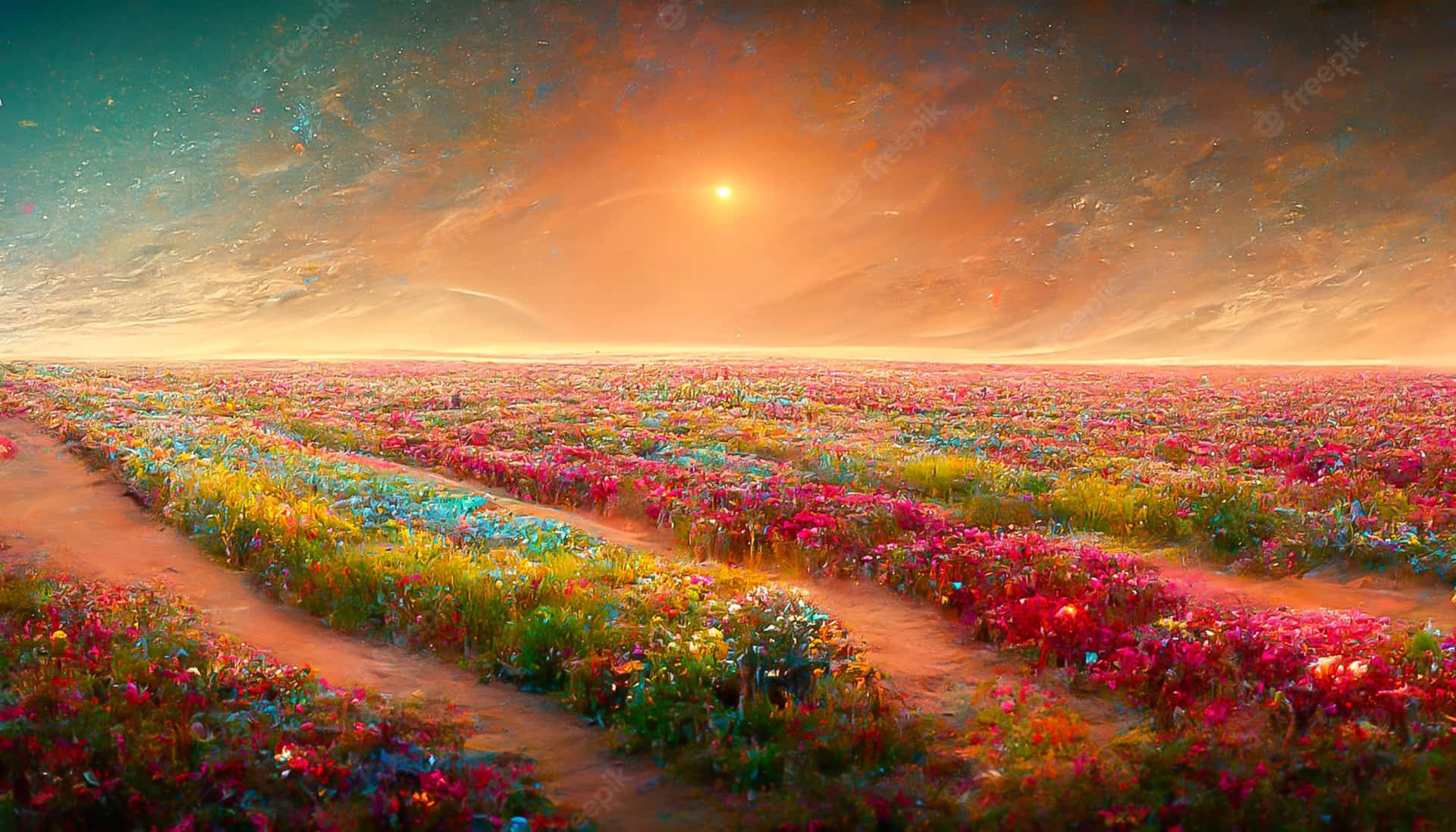This digital or painted artwork, available for download from the "freepick" website though copyrighted, portrays a vibrant and colorful field of flowers. The landscape format features rows of neon pink, neon blue, yellow, orange, and fuchsia flowers extending towards the horizon. Interspersed among the rows are identifiable walking paths that gradually blend and vanish into the continuous bloom as they stretch to the right. The sky in the painting is a striking gradient, with dark teal and deep blue hues to the left, transitioning into a radiant gold, amber, and salmon glow around the sun, before fading back into deep blues on the right. The sun, partially obscured by clouds, casts a warm golden light across the entire scene, enhancing the vividness of the flowers below. The overall ambiance of the piece is warm and colorful, with no human figures present, allowing the natural beauty of the landscape to take center stage.